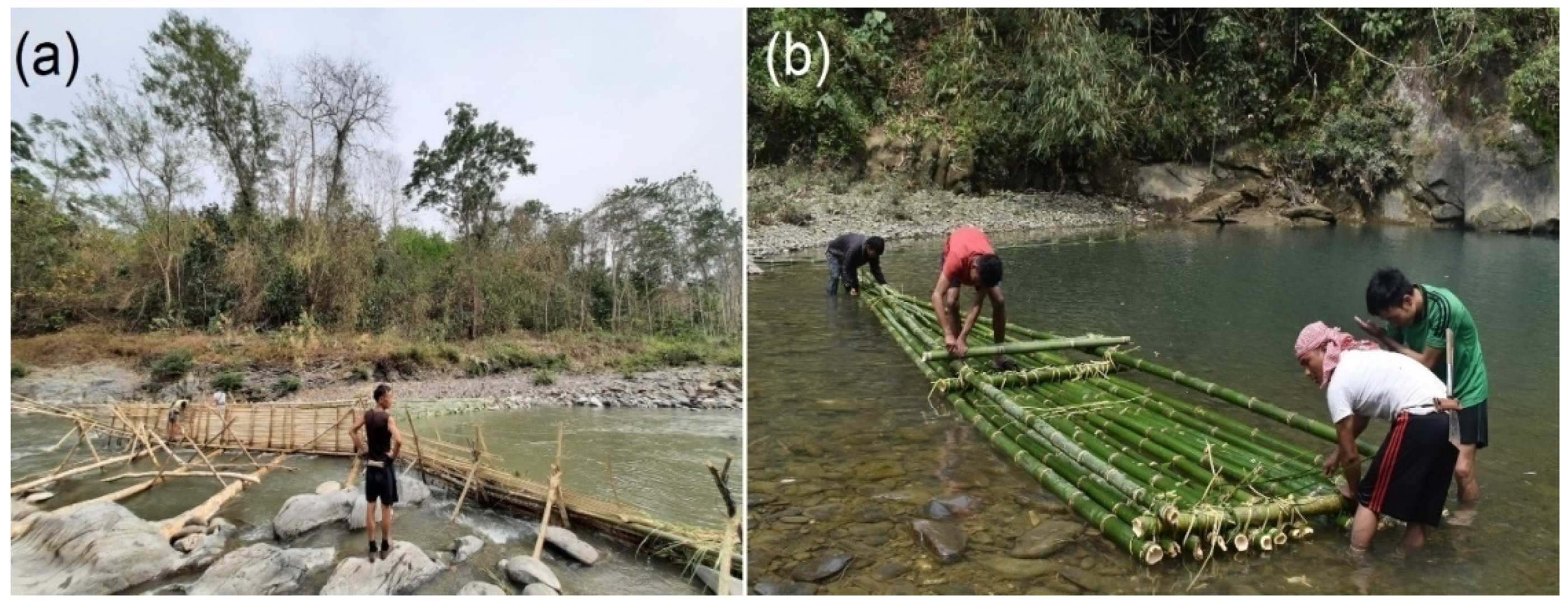The image depicts a side-by-side collage labeled “A” and “B,” showcasing two different scenes related to water and wooden constructions. In the left image labeled “A,” a solitary man stands on a rock in a river, near a makeshift bridge made from light-colored, balsa-like wood. This bridge appears fragile and rudimentary, not built to handle significant weight. The man, with hands on his hips, gazes distantly, surrounded by additional rocks in murky water. The scene features a grayish shoreline with sporadic green foliage in the background. In the right image labeled “B,” four men are knee-deep in the same murky water, collaboratively assembling a boat or a bridge from freshly cut, green bamboo shoots. They use a hay-like substance to secure the structure together. The bamboo construction seems more robust compared to the wooden one. The background is similarly dominated by a murky environment with grey and green hues, suggesting both scenes are set within the same location.